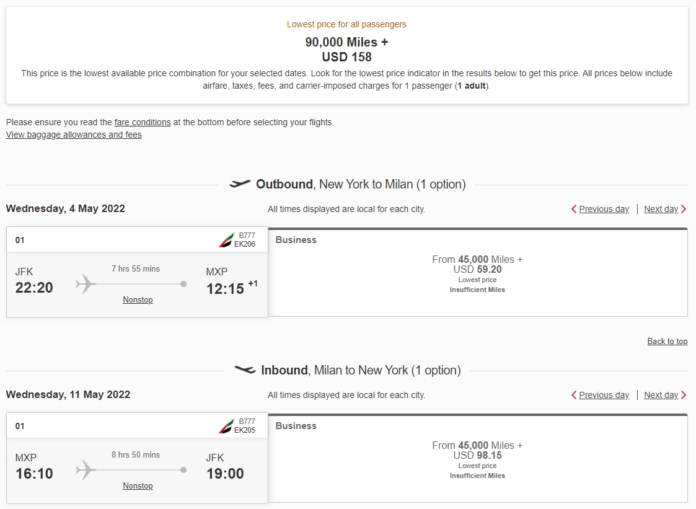Screenshot of the United Airlines website displaying the booking process for a round-trip flight from New York to Milan. The website has a prominent white background. At the top, in yellow text, it reads: "Lowest price for all passengers." Below that, it specifies in black text: "90,000 miles plus USD 158," followed by: "This price is the lowest available price combination for your selected dates. Look for the lowest price indicator in the results below to get this price. All prices below include airfare, taxes, fees, and carrier-imposed charges for one adult passenger. Please ensure you read the fare conditions at the bottom before selecting your flights. View baggage allowances and fees."

### Outbound Flight:
- **Route**: New York (JFK) to Milan (MXP)
- **Date**: Wednesday, May 4, 2022
- **Departure Time**: 22:20 (local time)
- **Arrival Time**: 12:15 (local time)
- **Class**: Business
- **Price**: From 45,000 miles plus USD 59.20

### Inbound Flight:
- **Route**: Milan (MXP) to New York (JFK)
- **Date**: Wednesday, May 11, 2022
- **Departure Time**: 16:10 (local time)
- **Arrival Time**: 19:00 (local time)
- **Price**: From 45,000 miles plus USD 98.15
- **Note**: Lowest price available, but insufficient miles.

This detailed caption accurately depicts the flight booking details, including dates, times, mile requirements, and additional costs.